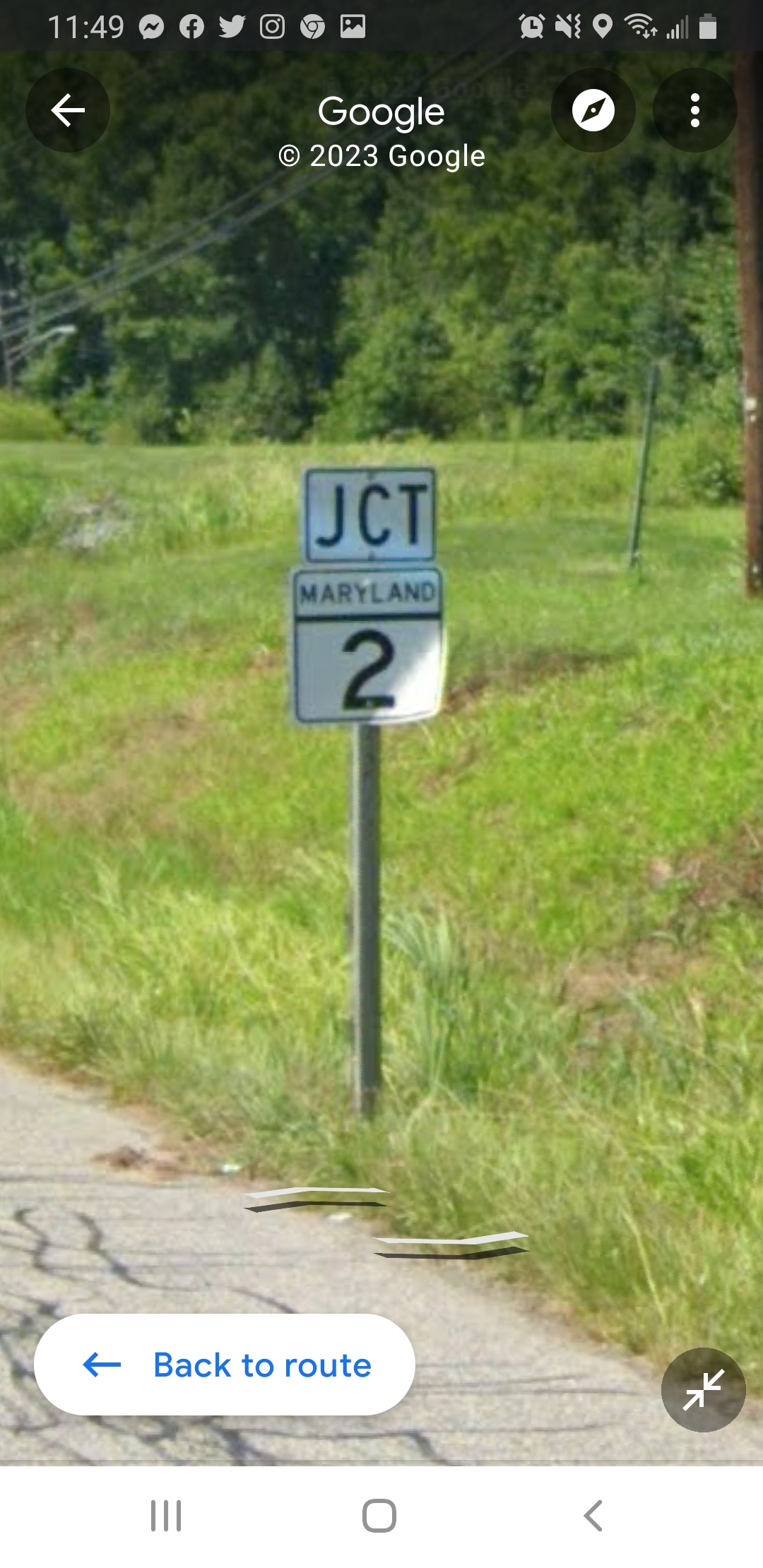This detailed caption combines the repetitive and unique elements each person mentioned:

A screenshot taken on a smartphone, displaying the time 11:49 at the top left. The taskbar at the top right indicates connectivity details, including Wi-Fi, signal bars, battery status, and various notifications from apps like Messenger, Facebook, Twitter, Instagram, Chrome, and an alarm icon, with the phone on silent mode. The screenshot appears to be of a Google image from 2023, as indicated by the text "Google 2023" and the copyright logo. The image itself features a green, overgrown grassy area with wild forestry in the background, broken concrete in the left corner, and a street sign on a silver metal pole that reads "JCT Maryland 2." There is a telephone pole with electric wires visible in the right corner, and two vertical cylinder-shaped objects located at the edge where the concrete meets the grass. At the bottom of the screenshot, a blue arrow links to 'Back the route.'